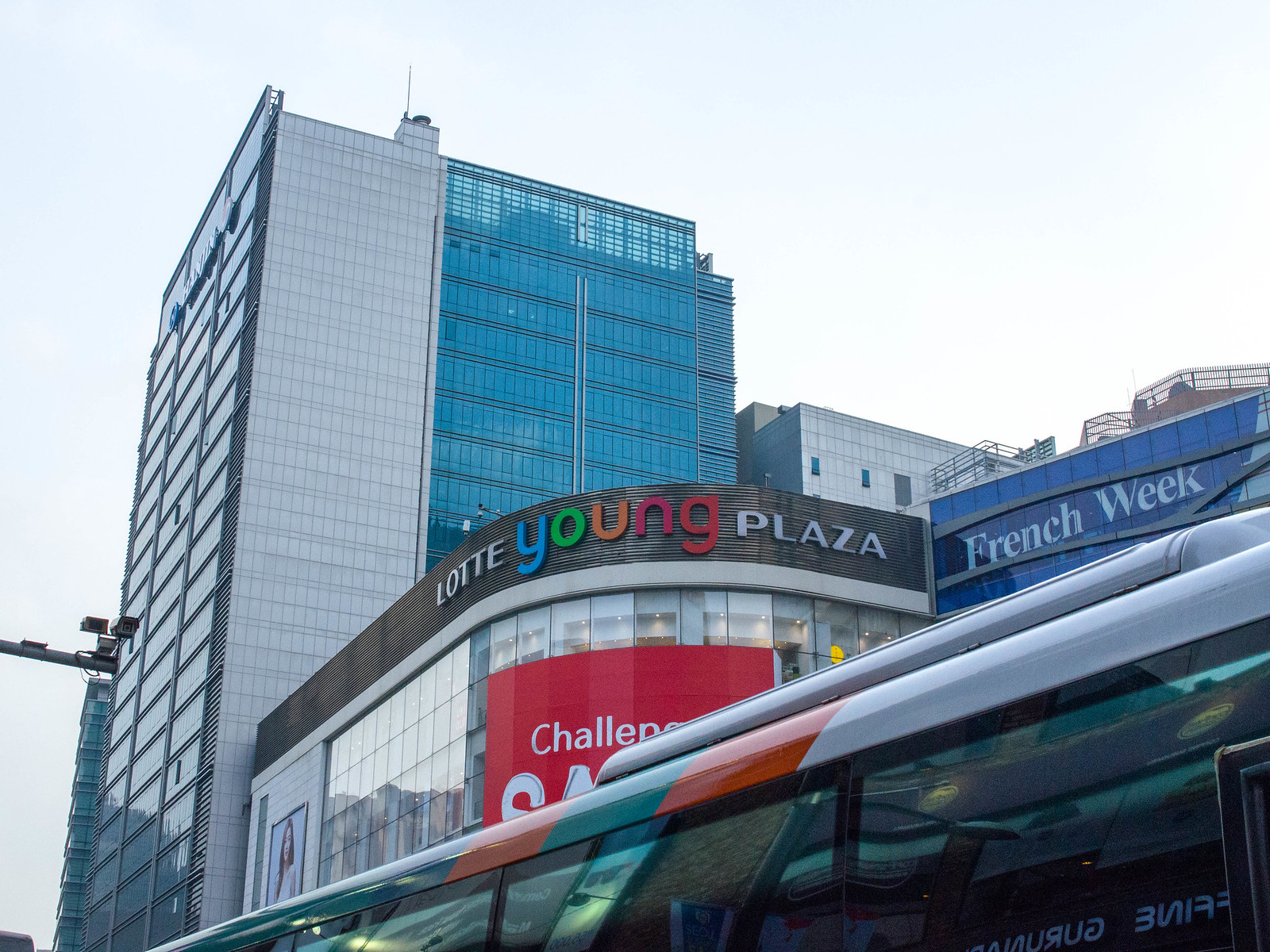The photograph is of an urban outdoor scene taken from street level, showcasing a bustling plaza on an overcast day. Dominating the image is the "Lotte Young Plaza" building, with its distinct sign: "Lotte" and "Plaza" in white lettering, and "Young" in a colorful gradient where each letter is a different color (Y in blue, O in green, U in orange, N in pink, G in red). The building's facade features a curved glass front, complemented by three windows on the left side and a white wall on the right. Below the "Young" logo, a red sign with white text reads "Challenge," though part of the text is obscured by what appears to be a bus or another structure in the foreground. Adjacent to the Lotte Young Plaza is another building with "French Week" displayed in white font. The scene captures a mix of modern architecture and urban life, with tall high-rises surrounding the plaza and contributing to the city's skyline.